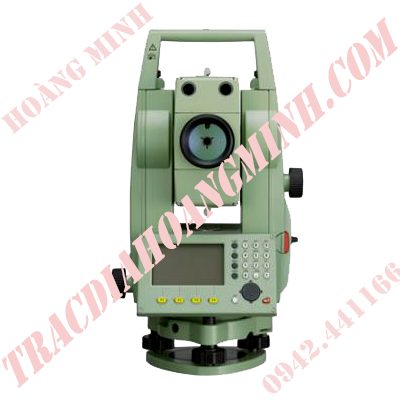The image features a detailed digitally rendered or possibly photographic depiction of a mint green, vertically-oriented machine placed centrally on a plain white background. This equipment includes a green handle at the top and several components: a black circular knob on its right side, a circular lens-like feature on the upper half, and two small black circles above it. Below these, there is a beige-colored digital screen flanked by four yellow buttons, and beneath that are four rows and three columns of small white buttons, with an additional large black button at the bottom. The device is elevated on short, black legs and features a noticeable watermark text. The watermark text, written in all-capital pink letters, says "HOANG MINH" diagonally across the top, "TRACKDIHONEMINH.COM" across the center, and the number "0942.441166" diagonally in pink at the bottom. The equipment and watermark suggest this image might be used in a stock image site or an online tool retailer platform. Colors present include white, pink, green, black, yellow, and red.